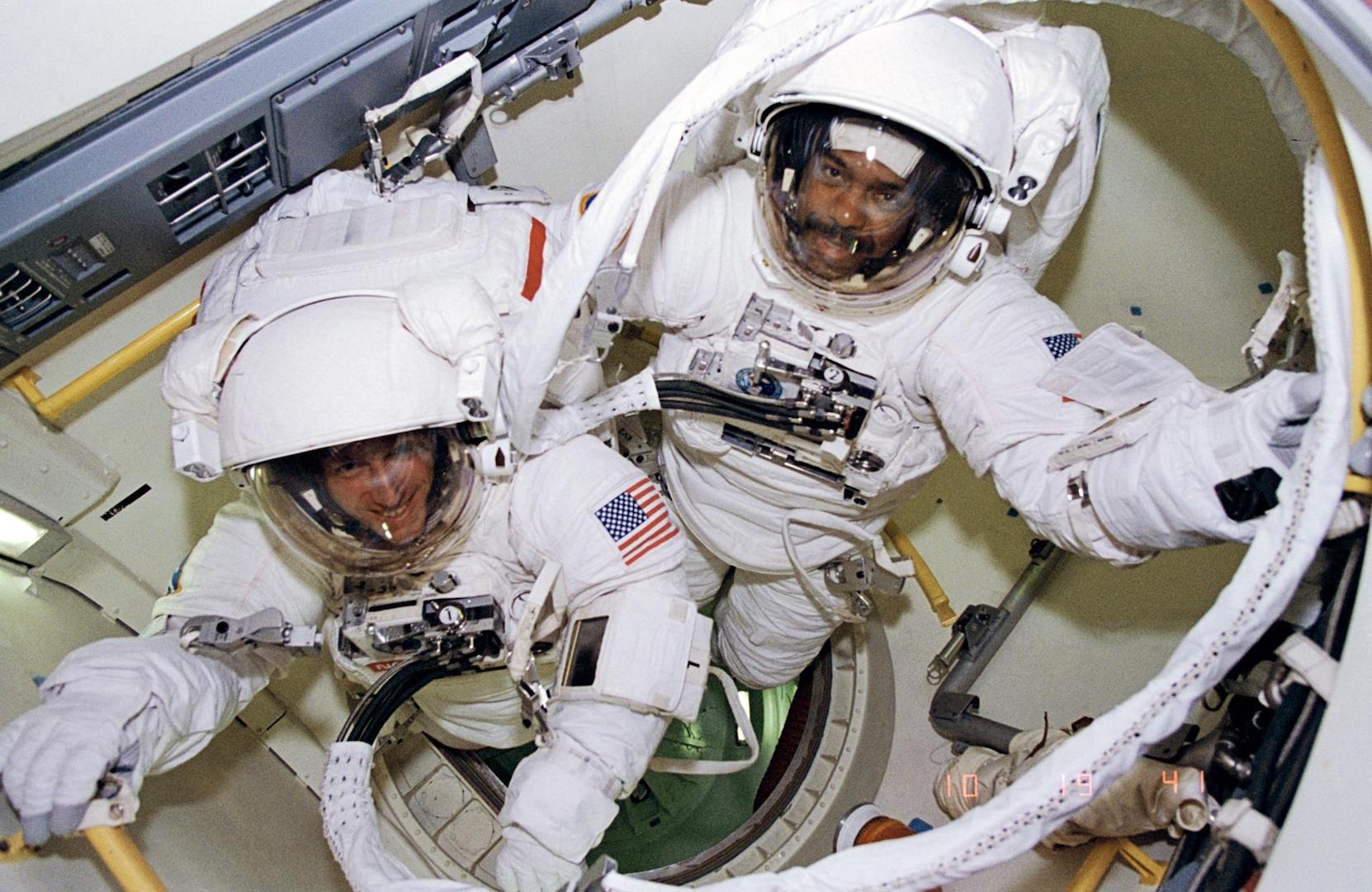This is a detailed photograph capturing two American astronauts in a confined space shuttle, seemingly floating in the weightlessness of space. The astronaut on the left is a white man, characterized by a wide smile and a tube emerging from his chest. This tube possibly connects him to the shuttle, indicating a work scenario. On his white space suit, along with white gloves and a helmet with a clear visor, the American flag is prominently displayed on his left sleeve. He's holding onto a ladder. His companion on the right is a black man with a mustache, also wearing a full space suit and appearing to look upward while floating through a circular porthole, suggesting a zero-gravity environment. He has a slight smile as well. A hose curls from the left astronaut's vest and snakes up towards the right astronaut's chest. They are surrounded by various machinery and components inside the shuttle, which are painted in shades of white and gray, enhancing the claustrophobic feel of the enclosed space.